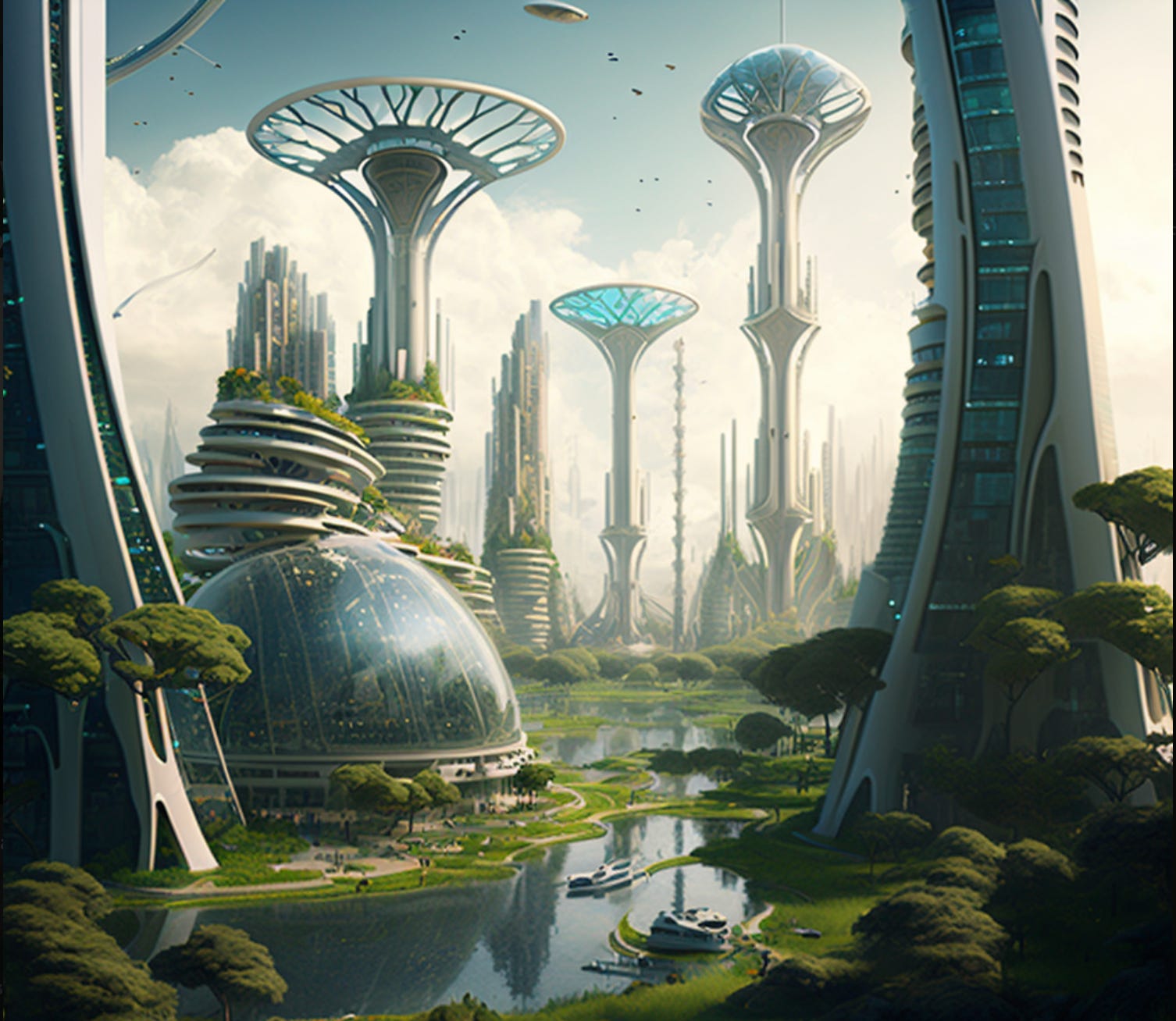The image is a detailed AI-generated digital artwork depicting a utopian futuristic city brimming with fantastical elements. Dominating the scene are towering skyscrapers shaped like trees and mushrooms, along with intricately designed multi-tiered layers adorned with lush greenery. The cityscape also features various angular bonsai-like trees and spherical structures, creating an otherworldly ambiance. In the lower left corner, a glass-domed building and jungle-like trees add rich complexity to the setting. A river weaves through the foreground, bordered by patches of grass and shrubs, while the air above is alive with flying ships and possibly flying saucers, contributing to the dynamic atmosphere. The city's skyline is filled with both tall, slender buildings with fan shapes and shorter structures with unique pipe segments. A twisting white building rises on the right side, while textures of blue iridescent glass domes and hazy skies complete the futuristic vision. Puffy white clouds reminiscent of a pre-thunderstorm sky enhance the scene's dramatic effect.